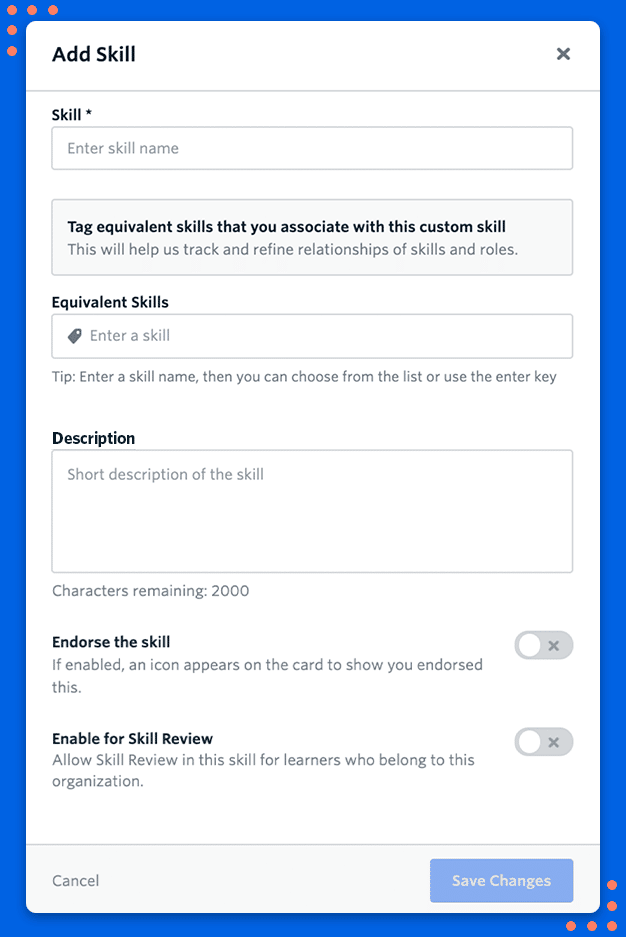The image features an interface on a blue background with orange dots in the top left-hand corner. A white pop-up box occupies the center, with distinct elements detailed as follows:

- **Header:**
  - "Add Skill" is prominently displayed in black at the top left of the white box.
  - A gray 'X' is located in the top right corner for closing the pop-up.

- **Skill Entry Section:**
  - **Label:** "Skill" with an asterisk indicating a required field.
  - **Input Field:** A box to enter the skill name.
  - **Tip:** In a gray box, it states: "Tag equivalent skills that you associate with this custom skill. This will help us track and refine relationships of skills and roles."

- **Equivalent Skills Section:**
  - **Label:** "Equivalent Skills"
  - **Input Field:** A box to input equivalent skills, accompanied by a tip beneath it: "Enter a skill name, then you can choose from the list or use the enter key."

- **Description Section:**
  - **Label:** "Description" in black.
  - **Input Field:** A text box for a short description of the skill.
  - **Character Limit:** It indicates "Characters remaining: 2000," specifying the limit for the description.

- **Options:**
  1. **Endorse the Skill:**
     - A toggle switch currently set to 'X.' If clicked, it enables an icon to show endorsement on the card.
  2. **Enable for Skill Review:**
     - A toggle switch currently set to 'X.' When enabled, it allows skill review for learners in the organization.

- **Actions:**
  - **Save Changes:** A button at the bottom right to save the entries.
  - **Cancel:** A button at the bottom left to cancel the action.

This thorough description covers each element in the interface, highlighting their functions and current states.